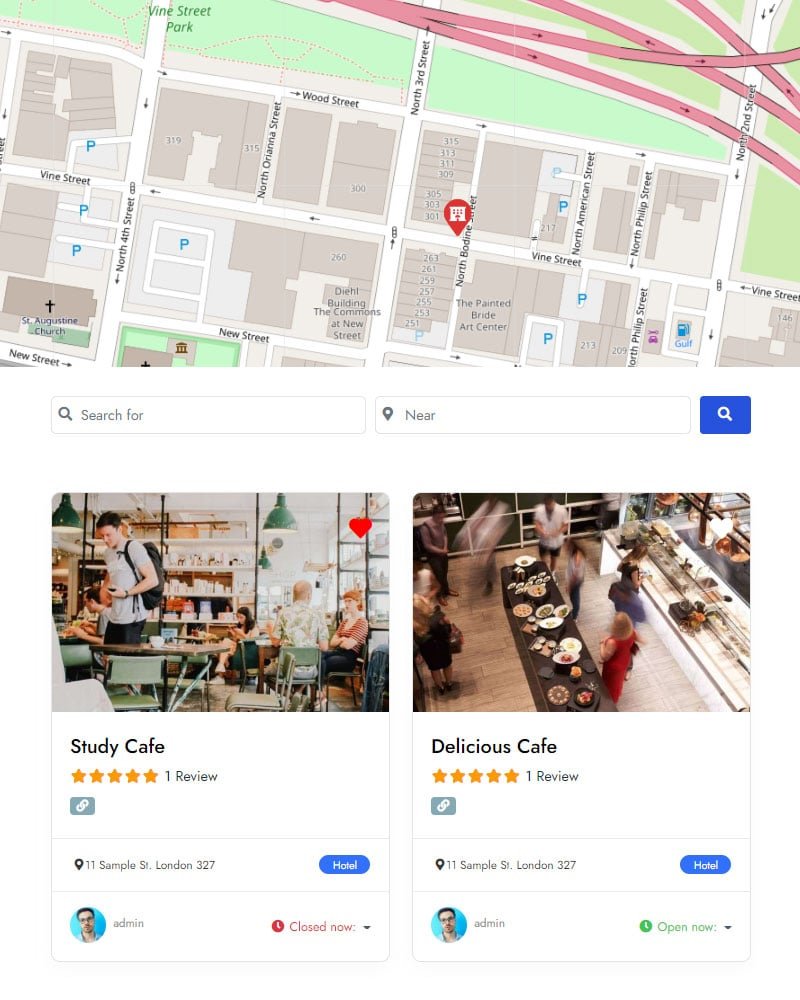The screenshot captures a map-based website interface. The upper half of the image features a 2D map highlighting streets, buildings, and roads with simplistic outlines. Green areas denote parks, while other regions are colored in tan and white shades. Directly beneath the map, there's a search bar allowing users to search for or select locations, accompanied by a blue search icon.

Below the search bar, two search results are displayed. On the left is "Study Café," which showcases a generic café image above its name. This café has received five stars from one review and is located at 11 Sample Street, London, 327. It is currently marked as "Closed Now," with the status displayed in red font.

The second result on the right is "Delicious Café," also depicted with a generic café image featuring people. It has similarly garnered five stars from one review and shares the same address: 11 Sample Street, London, 327. Unlike the Study Café, Delicious Café is described as "Open Now," with the status highlighted in green font.